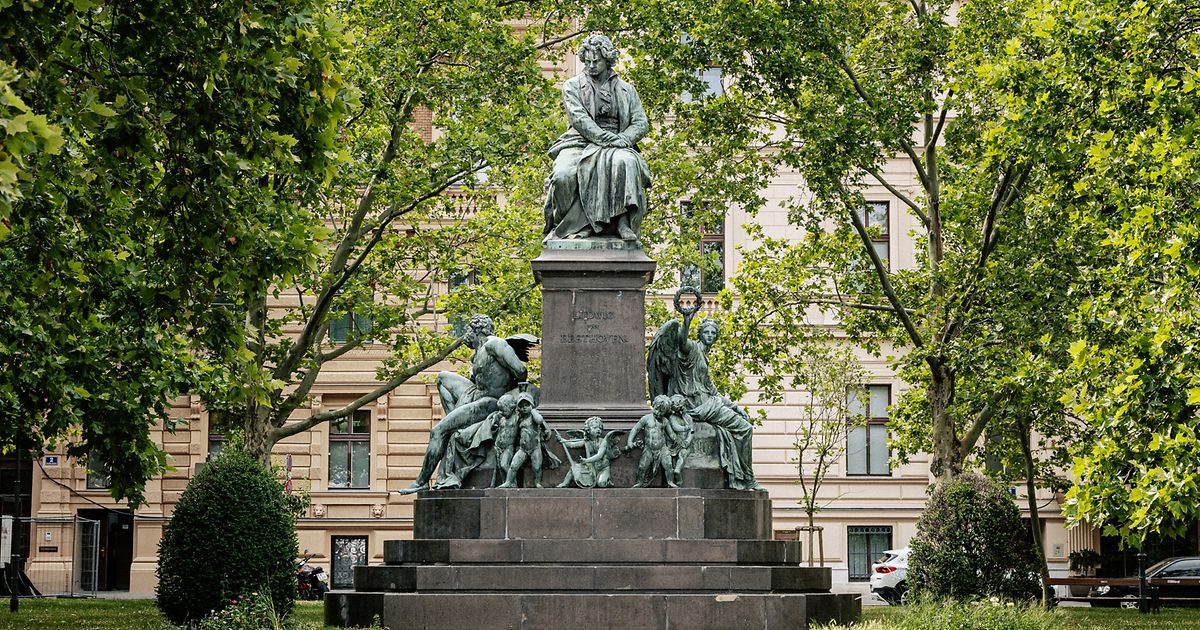This outdoor photograph captures a visually striking statue centered amidst a lush landscape. The statue, set against a light tan building with windows, stands on a four-tiered gray base. The lowest tier features five small cherub-like children with wings, semi-naked and playful. Flanking these cherubs on either side are two larger adult figures with wings, appearing to sit and each holding a symbol of importance, one with a crown. Rising above them all, a prominent statue of a man sits at the summit with both hands resting on one knee, gazing downward. The statue and its intricate details suggest a light blue, light gray hue. Surrounding this centerpiece are mature trees with dense green foliage, and small bushes are visible at the bottom. On the far right, there is an SUV partially visible, along with another brown car, adding a modern juxtaposition to the historic ambiance.